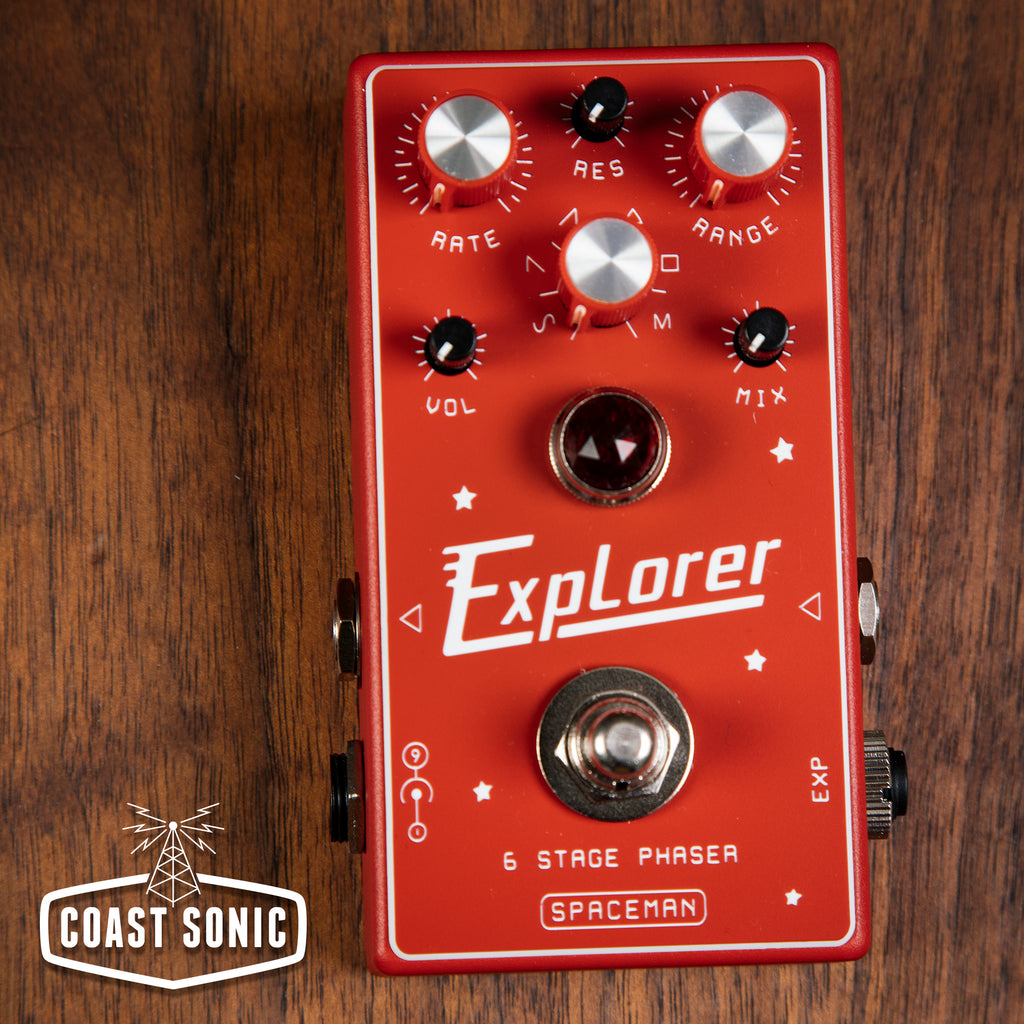The image shows a red electronic device, likely a phaser pedal for a guitar with various knobs and buttons used for live performance effects. The device is placed on a medium brown wooden surface. On the bottom left corner of the wood surface, a trapezoidal white outline encloses the text "Coast Sonic" in white, accompanied by a logo featuring an electrical pole with arcs of electricity.

The red pedal-like device prominently displays the word "Explorer" in white, with the "E" underlining the rest of the word. There are several labeled knobs and switches. At the top, from left to right, are silver and red knobs labeled "rate," "res," and "range," and black knobs with white lines labeled "volume" (abbreviated as "VLL") and "mix." In the center, there's a knob encircled by white and silver colors, featuring left and right arrows. Below this knob, an additional white and silver knob is present. The pedal also includes a small light indicator, currently off, and decorative elements such as white stars and left-facing arrows near the "Explorer" text. Additionally, the words “six-stage phaser” and "Spaceman" in white are situated near the bottom, along with a black knob marked with "EXP" in white.